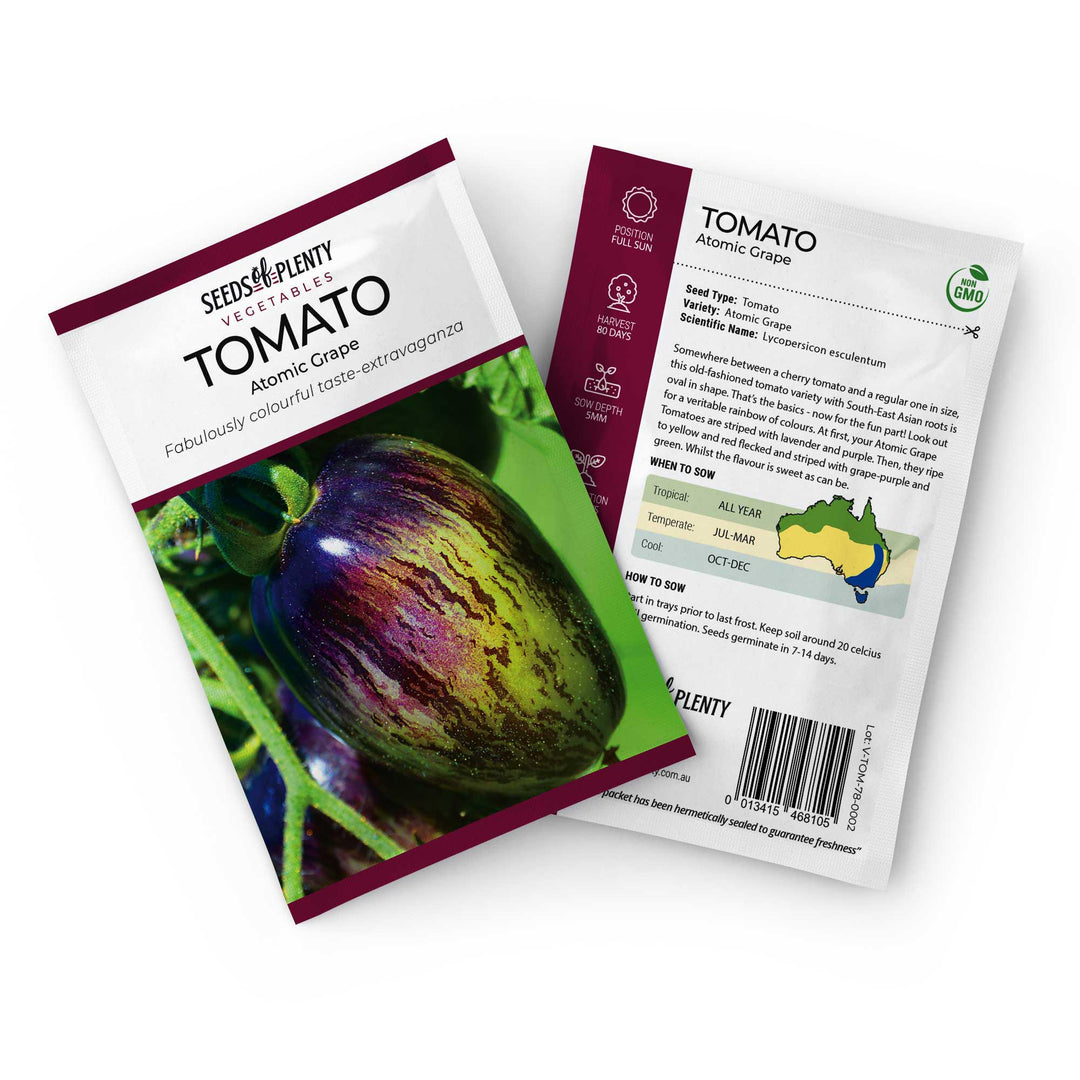The image depicts a seed packet for "Seeds of Plenty Vegetable Tomatoes," specifically the "Atomic Grape" variety. The front of the packet features a striking picture of an unusual tomato with green and purple streaks, attached to a green stalk. The front label reads: "Seeds of Plenty Vegetable Tomatoes, Atomic Grape, Fabulously Colourful Taste Extravaganza." The design prominently incorporates white and maroon (described as wine red), with maroon stripes on the top, bottom, and middle sections. In the background, green leaves are visible. The back of the packet, which is positioned underneath the front, carries a vertically oriented maroon design on the left side. It includes detailed information about the "Atomic Grape" tomato, non-GMO notice in the top right corner, and instructions for sowing. A barcode is located at the bottom right corner of the back.